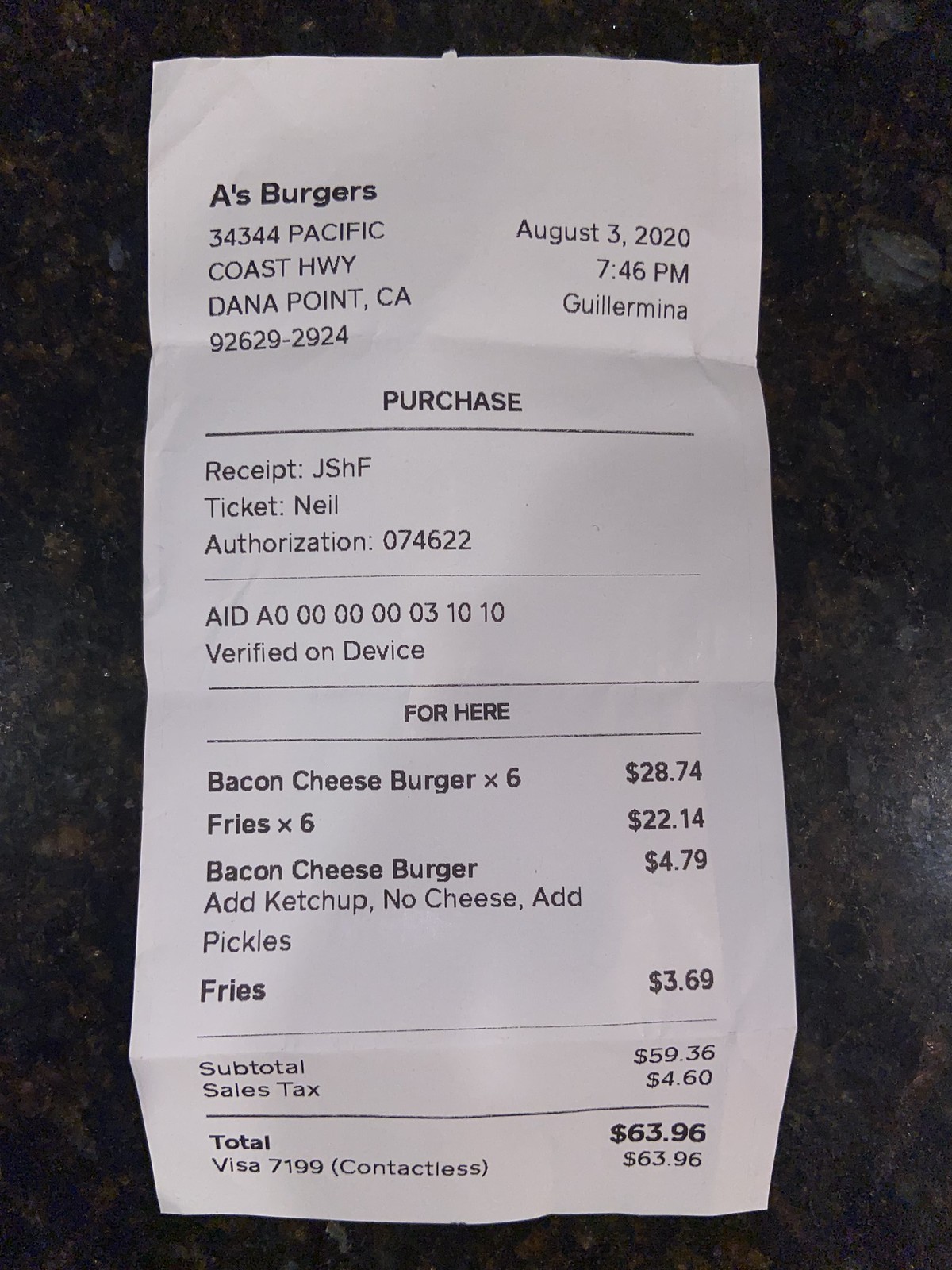In this photograph, we see a white rectangular receipt from A's Burgers resting on a black marble or granite countertop with subtle brown tones and visible smudges, coupled with a bit of light reflection. Details on the receipt include:

- Header: "A's Burgers" located at 344 Pacific Coast Highway, Dana Point, California, 92629-2924.
- Date and Time: August 3rd, 2020, at 7:46 PM.
- Server: "Gilermina" (spelled G-U-I-L-L-E-R-M-I-N-A) listed in the upper right.
- Purchases: Six bacon cheeseburgers at $28.74, six orders of fries at $22.14, an additional bacon cheeseburger for $4.79 with ketchup added, no cheese, and extra pickles, plus another order of fries for $3.69.
- Totals: Subtotal of $59.36, sales tax of $4.60, bringing the total to $63.96.
- Payment Method: Visa ending in 7199, with a contactless payment of $63.96.

The detailed receipt captures the essentials of a dining experience at A's Burgers, neatly printed on a used countertop's textured surface.